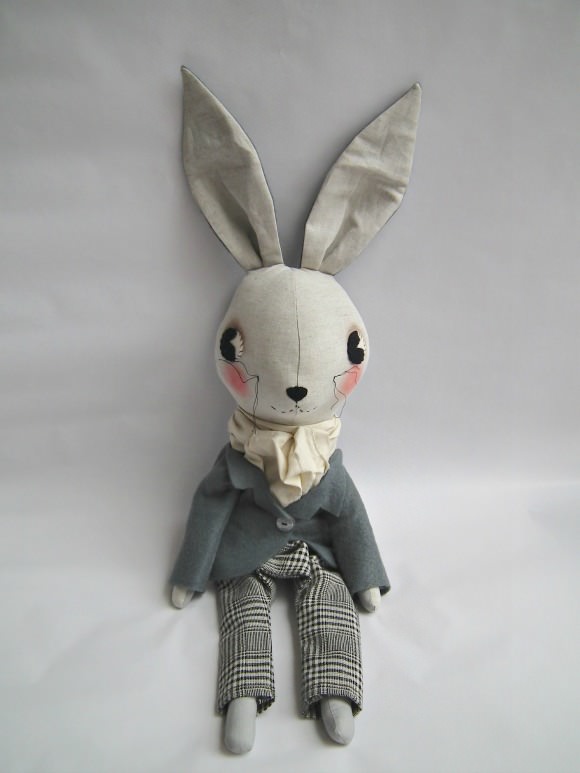This image features a meticulously detailed stuffed rabbit seated against a grayish white backdrop. The rabbit has a white, cotton or felt base with off-white linen ears, which are long and floppy. Its face is adorned with large, black eyes that have a bit of white detailing, rosy pink cheeks, a small black nose, and a dotted line for a mouth. The rabbit's attire exudes an old-fashioned charm, as it is dressed in a blue-gray sports coat over a frilly white shirt, resembling attire, possibly from another era. It wears distinct black and white striped or plaid pants, but no shoes. The hands and feet of the bunny are simply round, sewn ends of the limbs, lacking detailed paw features. The rabbit sits upright, presenting a solemn expression, making it a delightful yet nostalgic stuffed toy suitable for children.